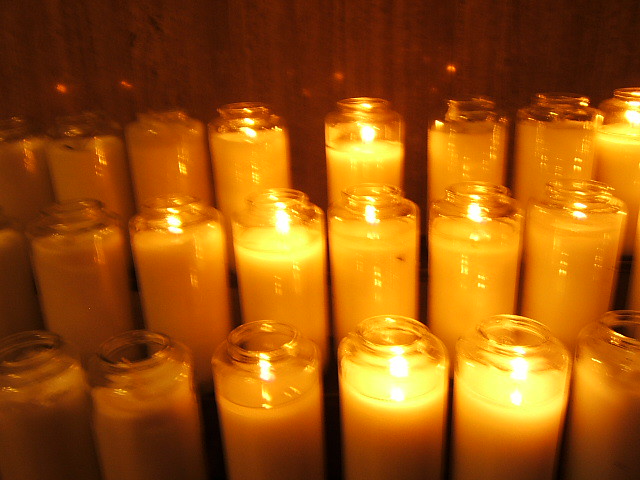This color photograph, taken indoors in a dimly lit room, showcases an array of candles housed in tall, clear glass jars, evocative of those found in a Catholic church. The image is oriented in landscape and features multiple rows of candles, meticulously aligned. The visible candles are organized into three horizontal rows: the top row holds eight candles with three lit, the middle row contains seven candles with five burning, and the bottom row consists of six candles, of which three are lit. The flame from the lit candles casts a warm, golden glow, creating an orange tint throughout the photograph. Reflections of the lighted candles can be seen against the dark brown, paneled wall in the background, adding to the serene atmosphere. Despite the subdued room lighting, the lit candles stand out vividly against their surroundings, offering a glimpse into what is likely a tranquil, contemplative setting.